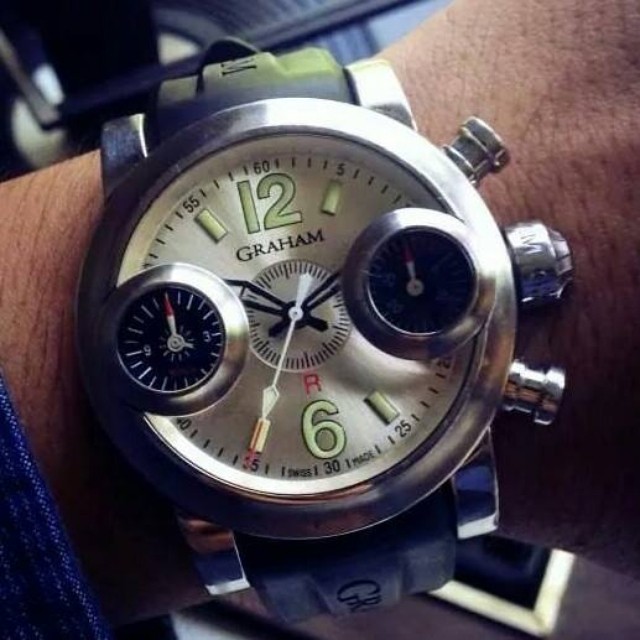This detailed close-up image captures a large, analog diver's wristwatch prominently displayed on a person's left wrist. The watch features a distinctive bronze-colored central dial, which is illuminated for visibility in low-light conditions. Unlike standard watches, this design only highlights the 12 and 6-hour markers, while the 3 and 9-hour markers are obscured by two smaller sub-dials that seemingly measure depth, a characteristic feature of diver’s watches. 

Made by Graham, the watch includes a band composed of a unique blend of blue and green rubber, providing both durability and comfort. The top section of the band appears green, while the bottom section seems blue. The background is blurred, offering little detail of the surroundings but focusing attention on the watch, suggesting the person is specifically showcasing their timepiece.